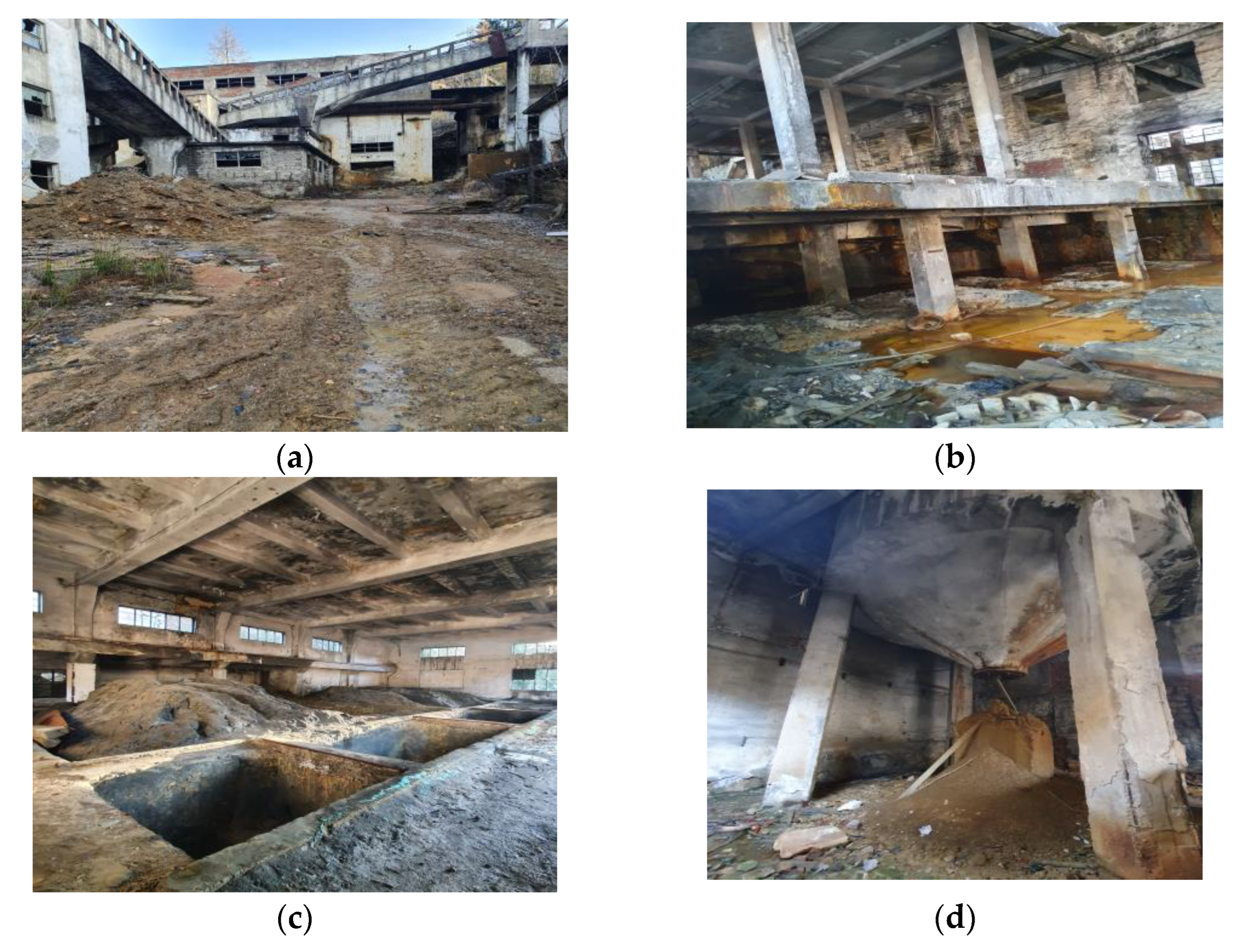This is a collage of four labeled photographs, A, B, C, and D, depicting an abandoned and deteriorated factory site, possibly subjected to flooding or natural disaster damage. 

Image A showcases the exterior of the facility, characterized by a muddy ground and a rusted conveyor system, with remnants of walkways or overpasses. The entire scene is dominated by earth tones—brown, gray, and yellow.

Image B offers a glimpse inside a dilapidated structure reminiscent of a parking garage, featuring deteriorated concrete pillars, scattered debris, and broken windows, all with a pronounced rusty discoloration.

Image C displays sections of the facility's interior with large rectangular pits or holes dug into a dirt-laden ground, surrounded by more evidence of structural decay and abandoned concrete beams.

Image D focuses on a large indoor milling or silo system elevated on concrete posts, with dirt accumulating below it and some kind of old containment bag or hopper. The pervasive sense of abandonment and disrepair links all images in this vivid portrayal of industrial ruin.